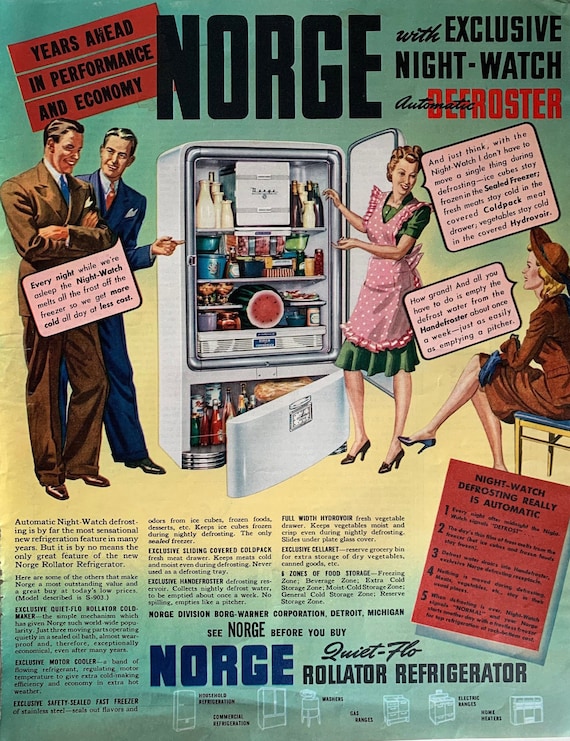This vibrant vintage advertisement illustrates a 1950s scene centered around a Norge Rolator refrigerator. The refrigerator, prominently open, showcases various items including drinks and a watermelon. In front of it, a smiling woman dressed in a green short-sleeved dress and a pink and white apron is pointing at the contents. She is wearing white heels. Seated to her right is another woman in a brown knee-length dress and matching hat, with blue shoes, sitting in a blue and wooden chair. To the left of the fridge, two men, one in a black suit and the other in a blue suit, converse with each other, both smiling. The background features a gradient of blue transitioning to yellow in the center, with captions reading, “Years ahead in performance and economy” and “Norge” in prominent red boxes. Other text highlights features like “zones of food storage” and “exclusive motor cooler,” and the description touts the fridge’s “night watch automatic defroster.” The bottom text invites viewers to “See Norge before you buy,” highlighting the refrigerator's innovative “quiet, flow, rollator” technology.